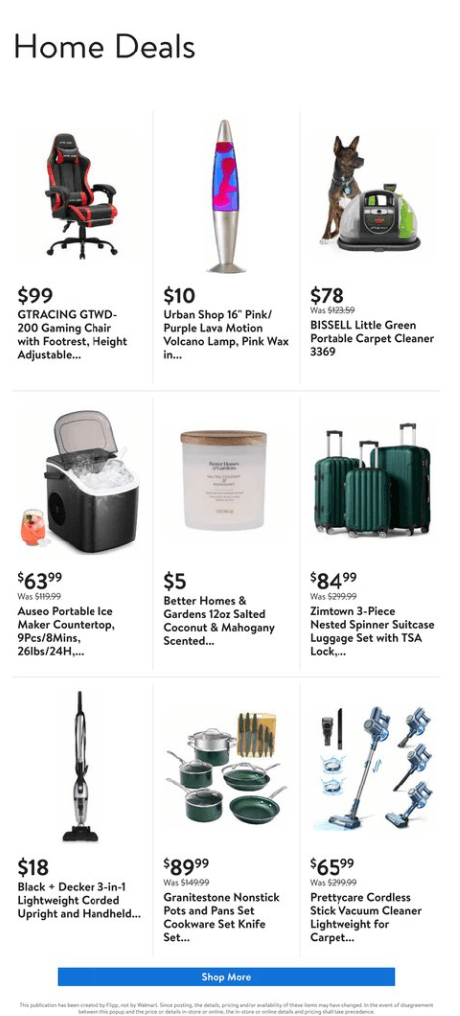This image depicts a sales page with a white background. At the top left corner, the text "Home Deals" is prominently displayed in black. Below this header, there are nine product images arranged in three rows of three.

- **Top left**: A red and black GTRacing gaming chair, priced at $99. It features a footrest and is height adjustable.
- **Top center**: A 16-inch Urban Shop pink and purple lava motion volcano lamp, priced at $10. Its wax appears to be pink.
- **Top right**: An image showing a dog next to a Bissell Little Green Portable Carpet Cleaner, priced at $78 (model 3369).

- **Middle left**: An RCO portable ice maker for countertops, priced at $63.99. It is black in color.
- **Middle center**: A 12-ounce Better Homes & Gardens coconut and mahogany scented candle, priced at $5. The candle is housed in a square container.
- **Middle right**: A set of three suitcases with handles, priced at $84.99.

This detailed layout helps viewers quickly identify and compare the products on sale.